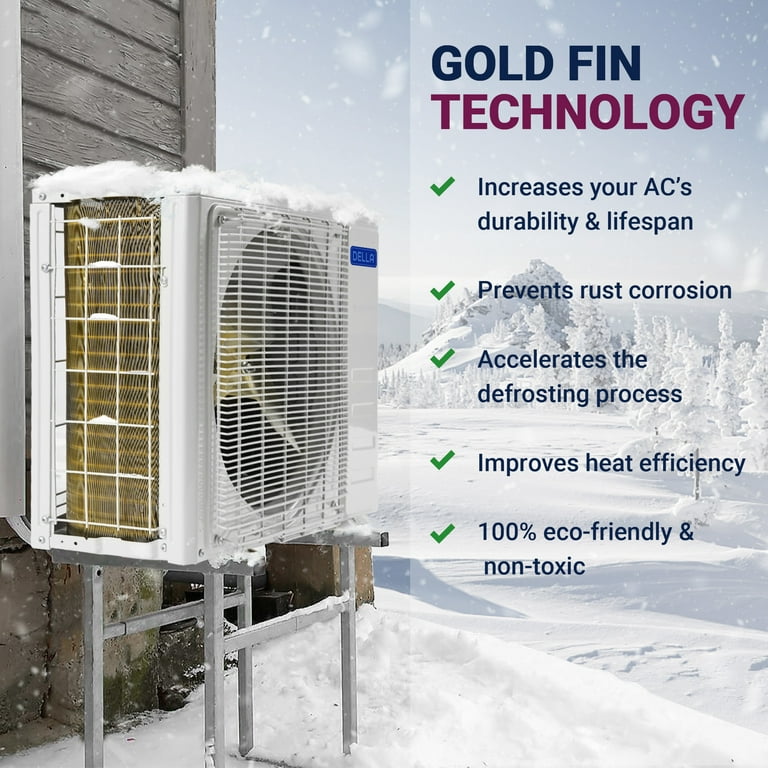The advertisement features Goldfin Technology, which is highlighted in bold blue and maroon letters on the right side of the image. Below this title, a list with green checkmarks details the benefits of this technology: increases your AC's durability and lifespan, prevents rust corrosion, accelerates the defrosting process, improves heat efficiency, and is 100% eco-friendly and non-toxic. The left side of the image showcases an air conditioner unit, identified as a Della, mounted on a silver framework against a gray wood wall. The unit, possibly a dual-function heat pump, is covered in snow and displays a gold-tinted grill with a visible fan blade inside. The backdrop features a snowy field with a tall hill and surrounding woodland, enhancing the wintry atmosphere with its white snow and blue sky color palette.